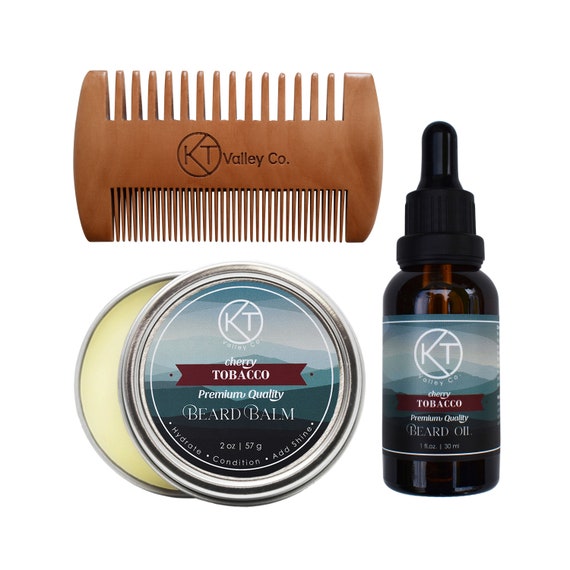The image showcases a detailed display of a beard grooming kit against a white background. At the top left, a brown wooden comb features two sides: one with widely spaced teeth and the other with closely spaced teeth. The comb is elegantly engraved with "KT Valley Co." Next, beneath the comb, stands a small aluminum jar labeled "Cherry Tobacco Premium Quality Beard Balm" with a capacity of 2 ounces (57 grams). This balm is designed to hydrate, condition, and add shine to the beard. To the right of the balm is an amber-colored glass bottle of beard oil, also labeled "KT Valley Company Cherry Tobacco Premium Quality Beard Oil." The bottle includes a dropper dispenser for precise application. The labels on both the beard balm and oil feature a bluish-white mountain depiction with white and red text highlights.